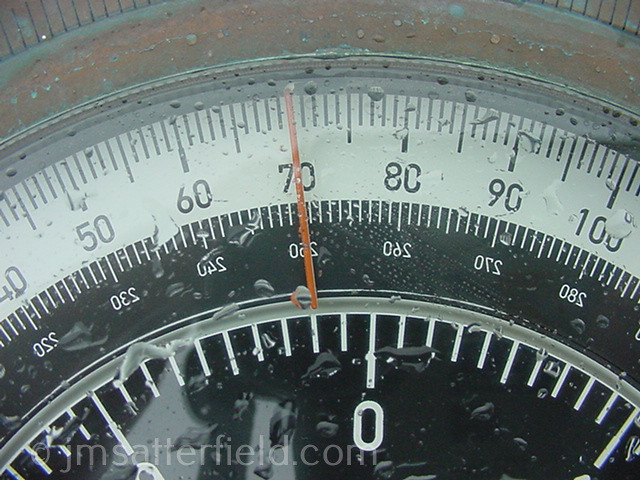Close-up of a scale's face covered in water droplets. The image captures the intricate detail of the droplets, emphasizing the texture of the scale's surface. The scale features an orange dial in motion, set against a white background with black numbers and markings ranging from 40 to 100, increasing in increments of 10. Directly below is a section with a black background and white markings, with numbers running in the opposite orientation from 220 to 280. Further down, another set of markings on a white background shows a visible zero. The backdrop appears to be a reddish, faded brick color. At the bottom, a semi-transparent gray text displays the copyright and website "jmsatterfield.com."